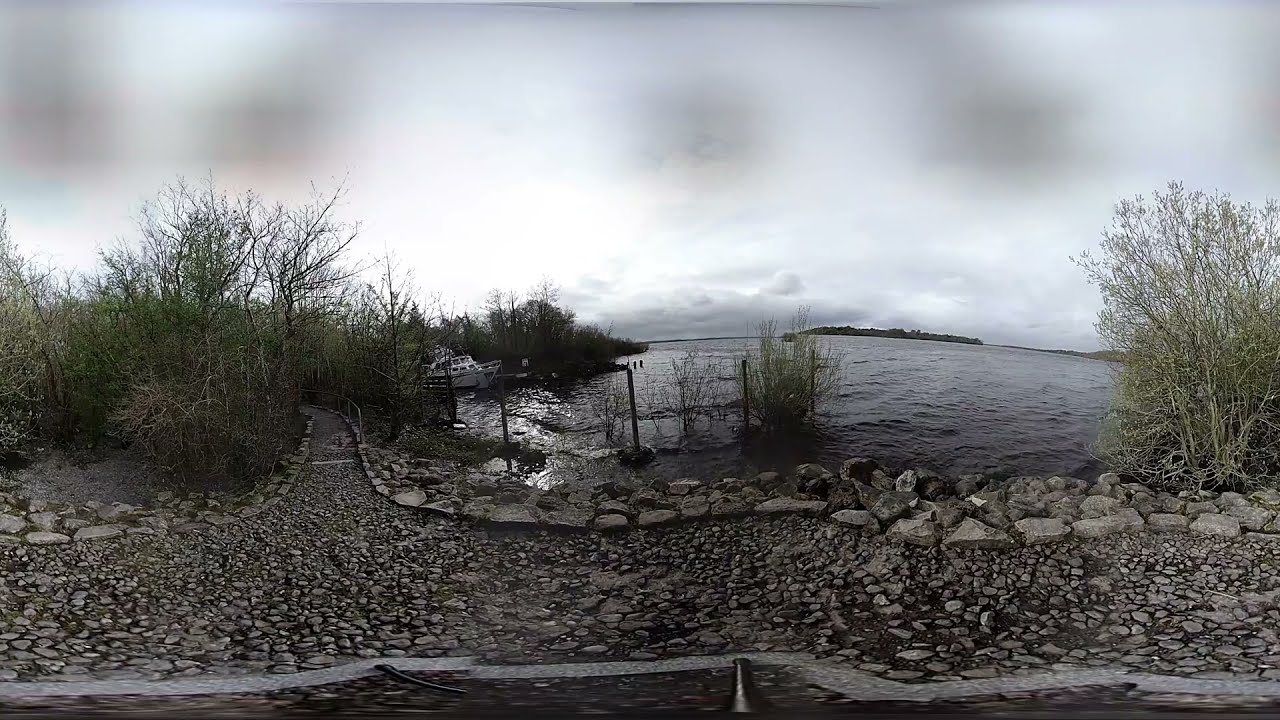This photograph captures a detailed view of a seashore landscape transitioning into a small bay or lagoon. Dominating the bottom of the image, the shoreline is composed of rocks and pebbles forming a rugged pathway. Along the shoreline, scattered plants and patches of seagrass add a touch of green, while remnants of a broken wire fence suggest bygone days of human activity. The shallow waters near the shore are clear, with additional sticks protruding from the water.

In the middle ground near the shore, a white motorboat, possibly a cabin cruiser or a fishing boat, is stationary, contributing a sense of human presence amidst the natural scene. The water, rippled by the wind, reflects shades of gray, indicating a breezy day. 

To the right, a distant landmass extends into the horizon, populated with trees, resembling an island or narrow piece of land. Centered further back, another landmass is barely perceptible against the meeting of water and sky. The sky above is a tumultuous mix of heavy, dark clouds, hinting at overcast weather or an imminent storm. The overall mood of the image is one of serene isolation, subtly touched by human influence yet dominated by natural elements.